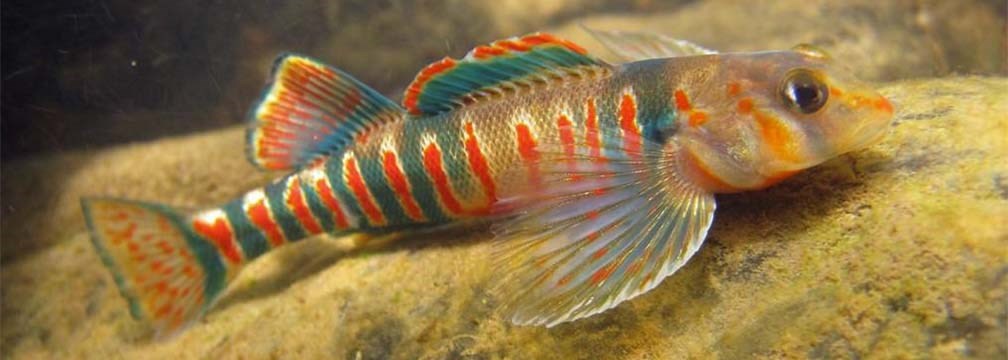A close-up, horizontally aligned, rectangular photograph captures a vibrant tropical fish, likely within an aquarium setting but possibly outdoors. The crystal-clear water reveals the fish resting on a pale yellowish-brown rock, with darker brown rocks visible in the upper left background. The fish, approximately finger-sized, boasts intricate and striking coloration. Its body features alternating bands of blue, gold, and reddish-orange stripes, with a diamond pattern of reddish-brown and light yellow scales. It has two clear side fins and gorgeously patterned top fins—orange-tipped with bands of green, brown, and blue. The rear fin exhibits orange and blue bands with yellow tips. Its tail is distinctive with a green border, a yellow tip adorned with orange markings, and spotted designs. The fish's head is partially clear with orange spots and a mix of tan, light yellow, and reddish-orange hues. Its singular dark brown to black eye stands out against its semi-translucent head. The backdrop suggests a faint light source illuminating the scene amidst surrounding darkness.